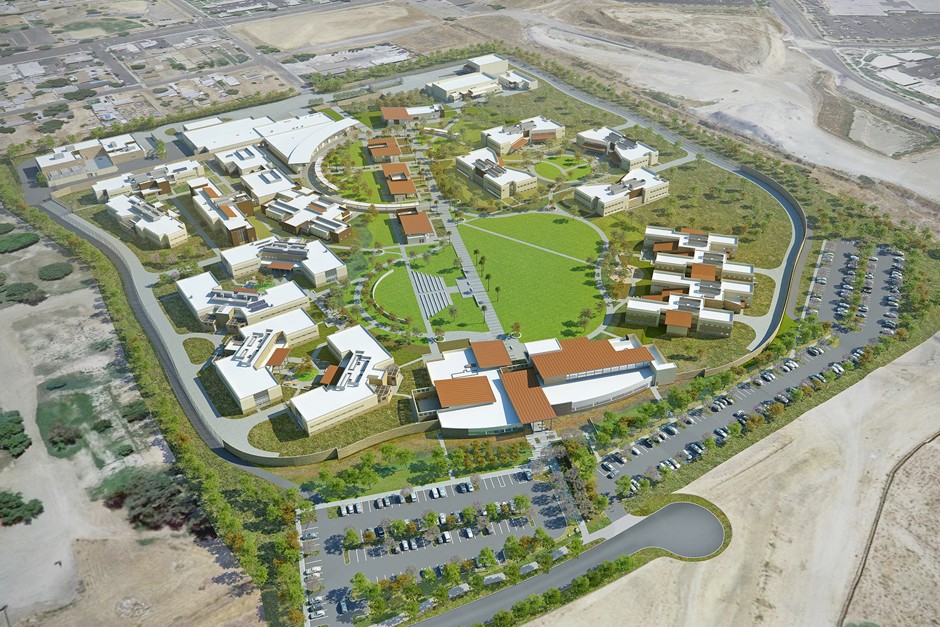This aerial view captures a sprawling small town or an industrial complex that blends urban and park-like elements. The image showcases a large, square plot of land dotted with a variety of building complexes and a centrally-located, well-manicured green area resembling a park. This central area features a flat expanse of lawn with steps and a long walkway, surrounded by lush, neat landscaping inclusive of trees and bushes.

Encircling this park are numerous buildings, distinguished by their roofs, which range in color from white to an orangish-brown hue. Towards the bottom of the image, an expansive parking lot stretches across the entire width, packed with around 100 cars. To the right of the park, three buildings are prominently visible, while the lower part houses a larger structure. On the left, there are four L-shaped buildings arranged in pairs, and a collection of smaller buildings with brown roofs situated behind the park area.

Sidewalks and walkways weave through the complex, accompanied by meticulously maintained landscapes, giving the whole area a planned and organized aesthetic. This bird’s-eye perspective, likely from a helicopter or airplane, offers a comprehensive view of this attractive and functional space designed to support a bustling hub of activity or workplaces.